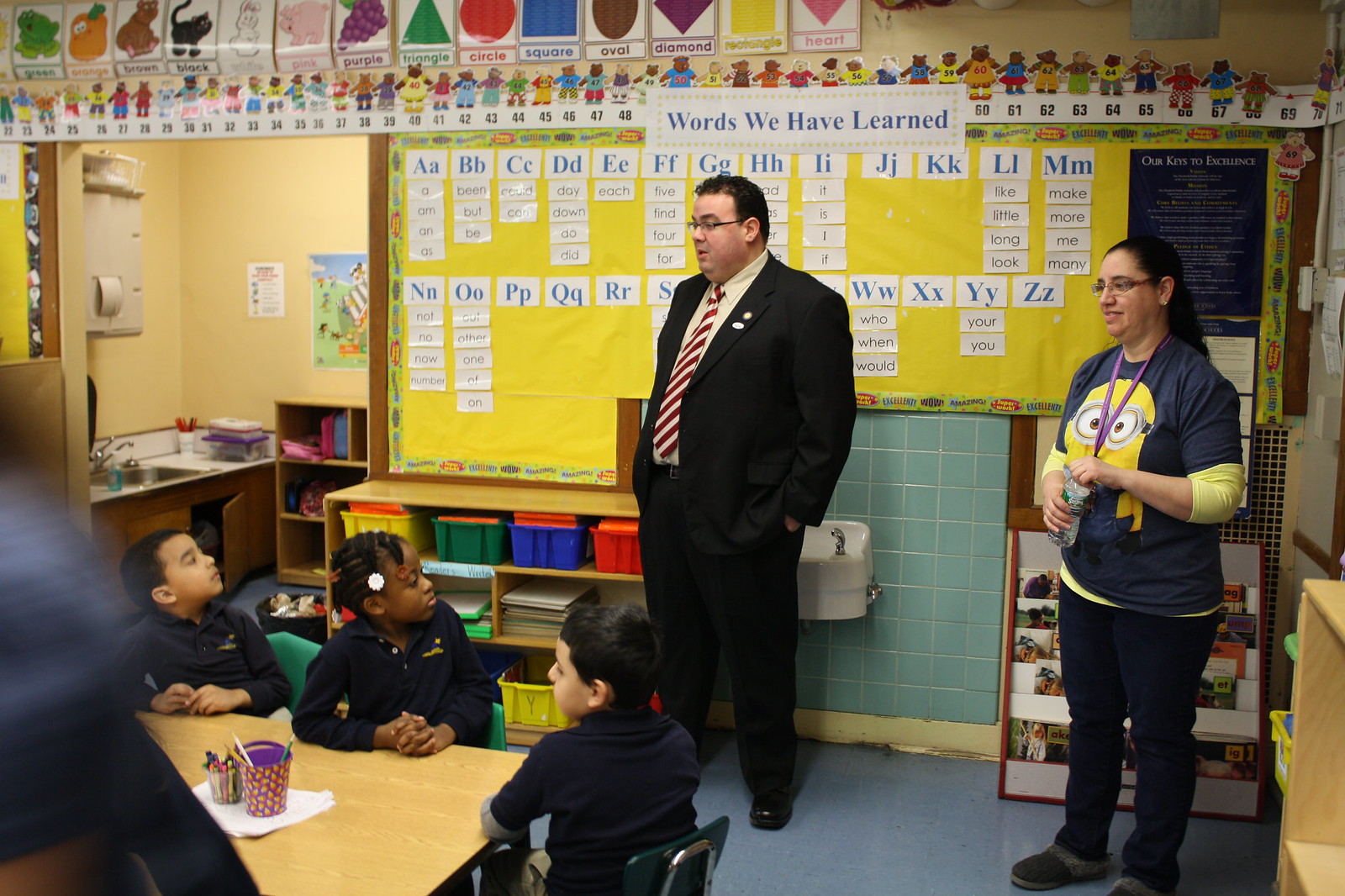This image captures a lively classroom scene set indoors, likely in the middle of the day. The focal point is a group of young children, possibly kindergarten-aged, sitting around a brown table in the lower left corner. The children appear to be of diverse ethnic backgrounds and are wearing blue polo shirts. On the table, there is a cup filled with crayons, another with pencils, and a cup decorated with candy corns.

At the center of the image stands an overweight man in a black suit with a white shirt and a candy cane-striped tie, addressing the children. He is wearing glasses and his hands are in his pockets. To the far right, there is a female teacher, identified by her Minions t-shirt worn over a long-sleeve shirt and a lanyard around her neck. She appears to be opening a bottle of water and is smiling at the scene.

The classroom is richly decorated: the back wall features a banner with the words "Words We Have Learned" organized alphabetically, accompanied by various letters. Above, a colorful border displays shapes (triangle, circle, square, oval, diamond, rectangle, heart) and colors (including green, orange, brown, black, white, pink, purple, and yellow) with corresponding examples such as a pink pig. The room also has educational material like cubbies, a drinking fountain with a blue tile backdrop, and a low-hanging ceiling with numbers and additional educational decorations. The flooring in the classroom is linoleum, adding to the typical school environment ambiance.